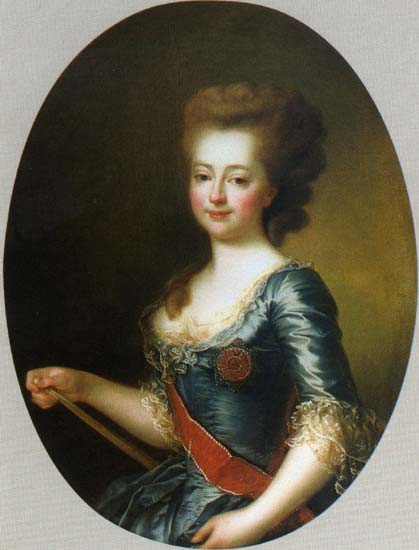This image features a detailed painting of a woman, prominently positioned within an oval frame that itself is enclosed by a rectangular frame. The rectangular frame, although primarily obscured, reveals its gray background at the corners. Dominating the image is the oval frame, which houses an intricate depiction of a woman dressed in what appears to be a blue Victorian-style dress. The dress is elaborately designed with ruffled sleeves, approximately elbow-length, and accentuated by a red sash crossing the midsection and a distinctive red circle on her left breast. She has a pale complexion, highlighted by rosy red cheeks, red lips, and a touch of redness on her nose. Her reddish, or perhaps brown hair, is styled in an old-fashioned manner, cascading down her back and over her right shoulder. She gazes forward with a subtle, small smile, her blue eyes giving her a serene yet regal appearance. Her right arm is extended to the left, holding a stick-like object, while her left arm rests at her side. The background within the oval frame presents a simple brown wall, further drawing attention to the detailed portrait. The painting bears no signatures or text, leaving the identity of the woman, who resembles a figure of nobility or possibly a queen, shrouded in mystery.